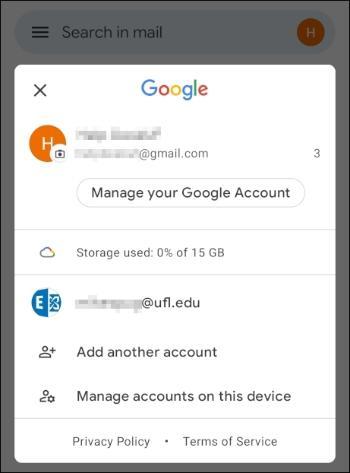The image is a screenshot of a mobile device displaying the "Accounts" section within the device settings. The focus is on the Google account and other accounts, both of which are shown in a grayed-out state. Text elements on the screen include "Manage your accounts" and "Storage used: 0% of 15 GB." Options such as "Add another account" and "Manage accounts on this device" are also visible. Towards the bottom of the screen, links to the "Privacy Policy" and "Terms of Service" are provided. The background of the interface is white, with black text for readability. Additional colors present include orange and blue, providing a minimalist yet functional design. At the top of the screen, there is a search bar labeled "Search in mail field," indicating the potential for quickly navigating email content.